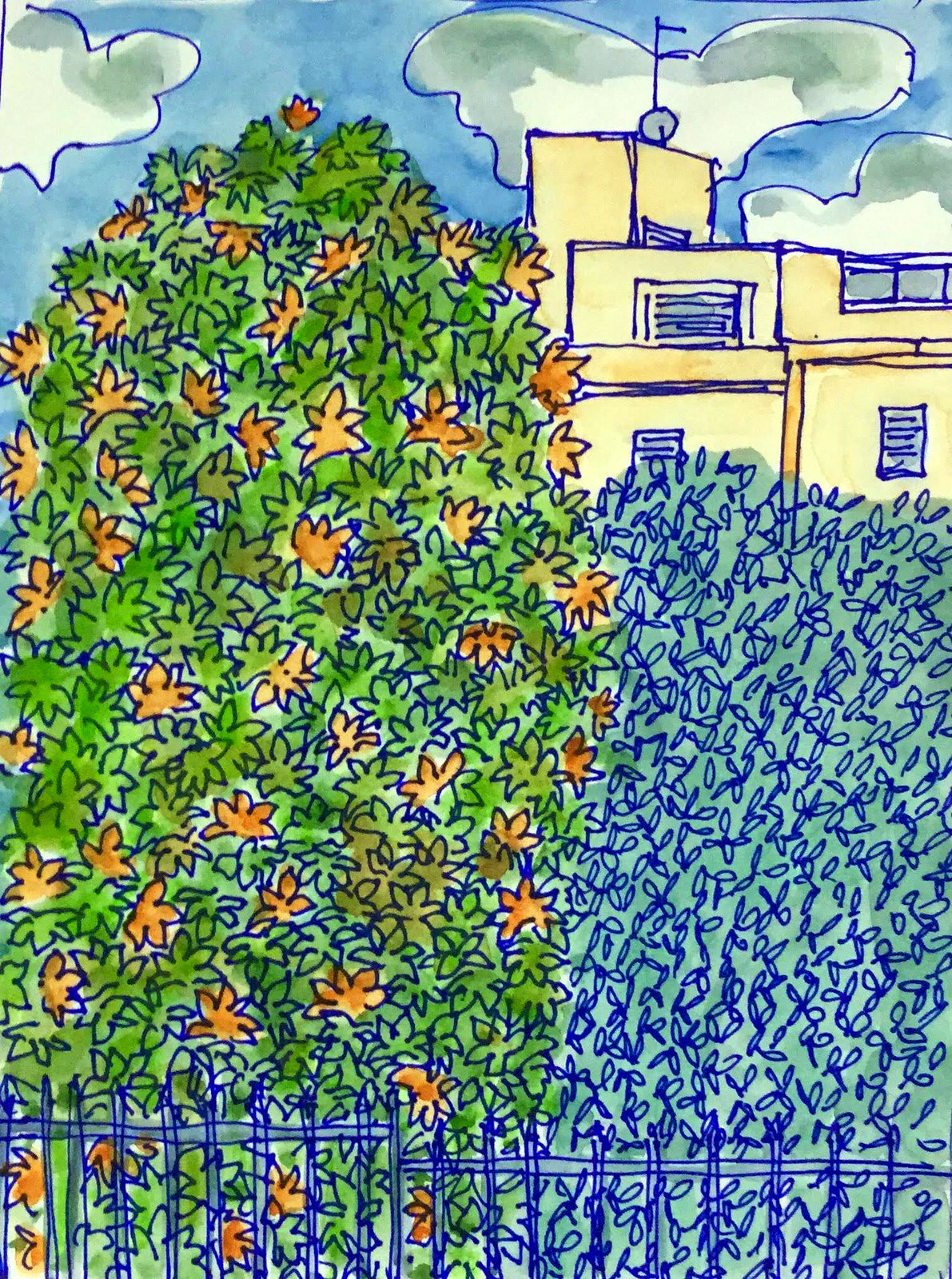In this intricate drawn image, the eye is first drawn to the bottom where a blue pen outlines a gate, filled in with a light blue shade. On the left side, a large, lush bush dominates, nearly reaching the top of the image. This bush is predominantly green, with touches of orange, yellow, and brown leaves scattered throughout, adding depth and texture. Meanwhile, on the right side, a smaller shrub-like object stands out with its light green hues. The top right corner features a multi-level yellow building capped with a satellite dish. This structure contrasts sharply with the vibrant elements surrounding it. The backdrop of the image is a serene blue sky, adorned with numerous curvy cloud-like shapes, white with grey shadings, contributing to a dreamy, whimsical atmosphere.